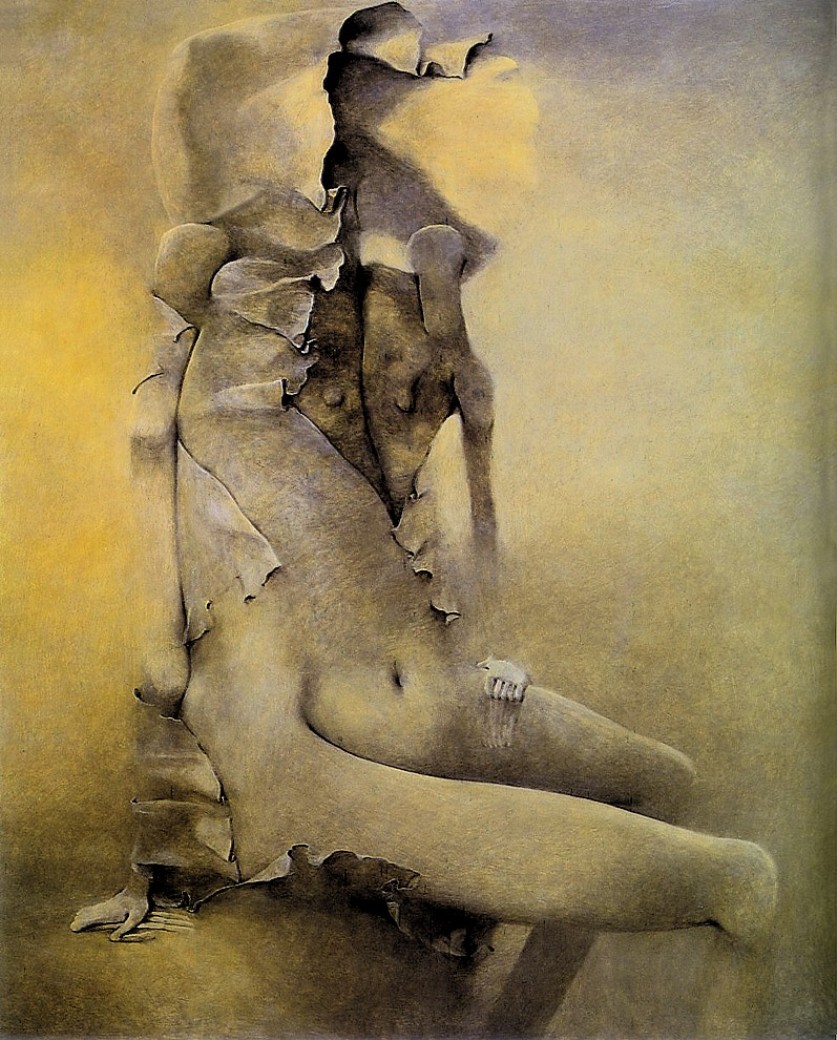The image is a highly detailed, surreal drawing with an emphasis on pencil shading, featuring primarily black and tan hues. The scene depicts a disjointed, feminine figure transitioning into a state of decay. The figure appears to be emerging from or wrapped in a fabric or paper sheet-like material. The upper part of the figure includes a chest that is opening up, revealing a face inside, while the head is conspicuously absent, replaced by a hood-like form. The chest area is exposed, showing two nipples. The right side of the figure's body is particularly skeletal; a prominent hand on this side reveals bone structure. On the lower part of the image, the legs are positioned unusually high, showing a belly button, and one of the hands, with six fingers, grips the left leg. The overall composition is muted, detailed, and haunting, combining elements of decomposition with abstract fabric forms.